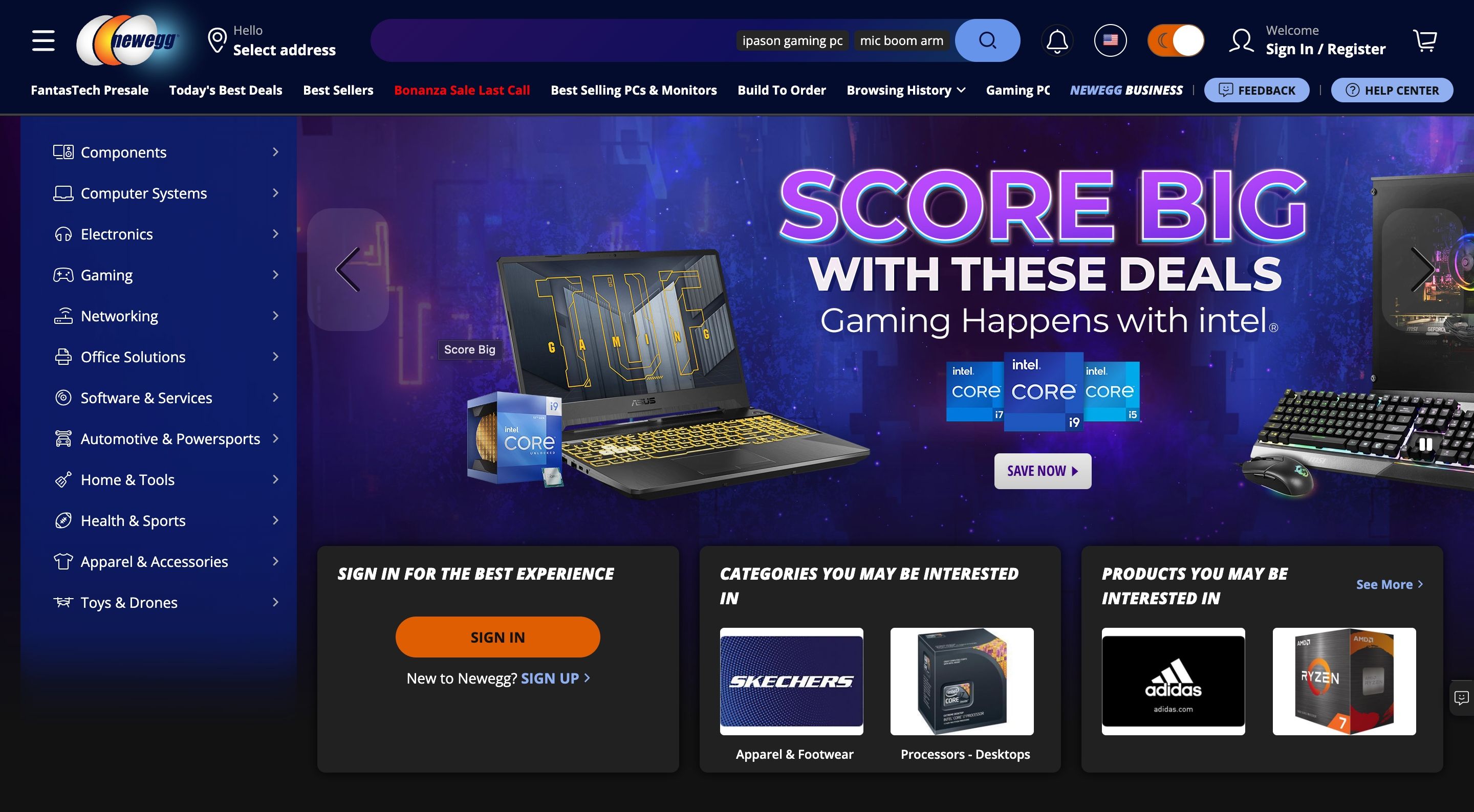Here is a detailed and cleaned-up caption for the image:

"This is a cropped screenshot of the Newegg.com home page, specifically the desktop version. The top left corner features a dark blue background with the Newegg logo displayed. Adjacent to the logo is a white menu icon. Following that, there is a location pin icon, succeeded by a small white text saying 'Select Address,' which allows users to choose a store address. Next, a search bar occupies the space with two suggested searches, 'gaming PC' and 'mic boom arm,' followed by a light blue search button. To the right of the search bar are a series of icons: an alert icon, an American flag icon indicating the site's language setting, and a toggle switch for dark mode with a moon icon. Further right are the sign-in/register icon and a shopping cart icon.

Below this top bar, there is a horizontal menu with various options, displayed in small white letters. On the far right of this menu are two blue buttons labeled 'Feedback' and 'Help Center.' 

On the left side of the page is a vertical panel featuring different categories, each with an icon, category name, and an arrow pointing left, indicating expandable sections.

The central part of the page displays a promotional banner with a background image of two angled computer setups. Across the center of the banner, large purple text reads 'Score Big,' with smaller white text below saying 'with these deals.'"